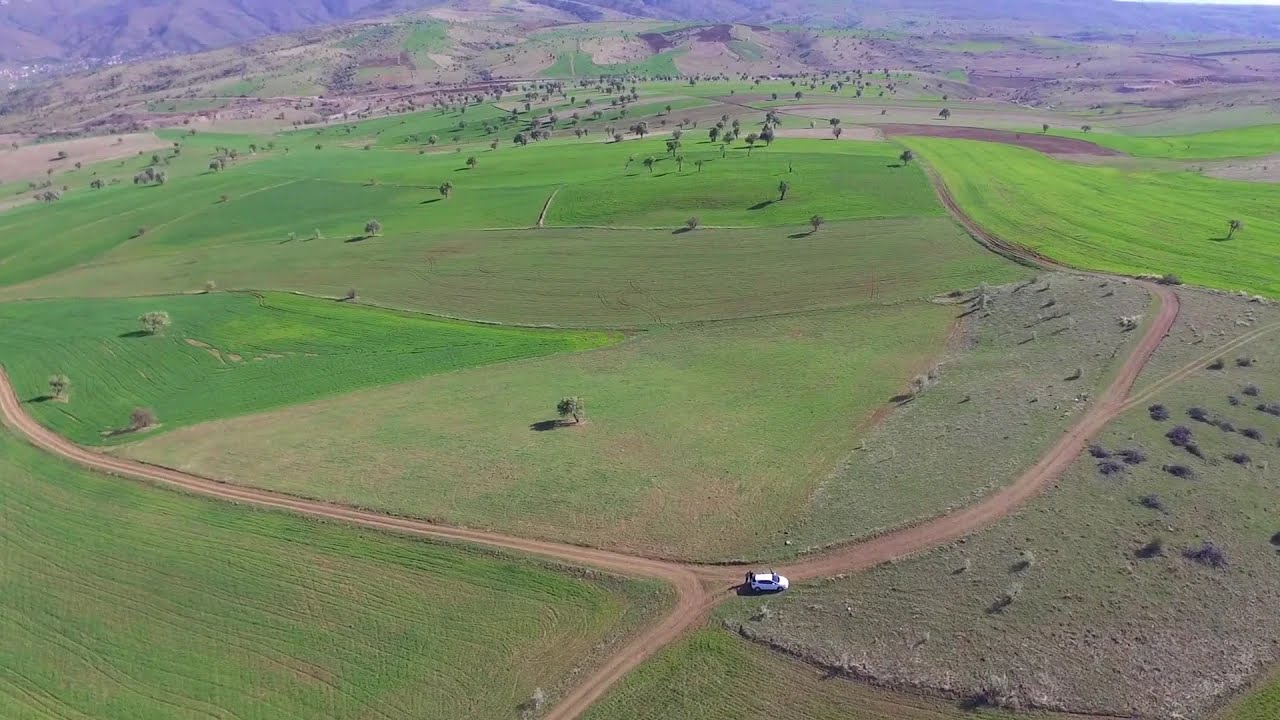The image, captured via drone, portrays a vast landscape featuring a vibrant, green expanse segmented into different sections of grass ranging from dark to lime, with some areas appearing slightly worn. This green grassland is interspersed with widely spaced trees, leading the viewer's eye towards a distant range of hills and mountains. In the foreground, a dirt road winds through the scenery, with a white car traveling along its path and at one point appearing parked at a section of the road. The road curves and branches off, creating various routes across the landscape. The scene is bathed in daylight, with the sun highlighting the contrasts between the different shades of green and the patches of dirt. The overall effect is reminiscent of a whimsical, almost storybook-like setting, merging natural beauty with rustic charm.